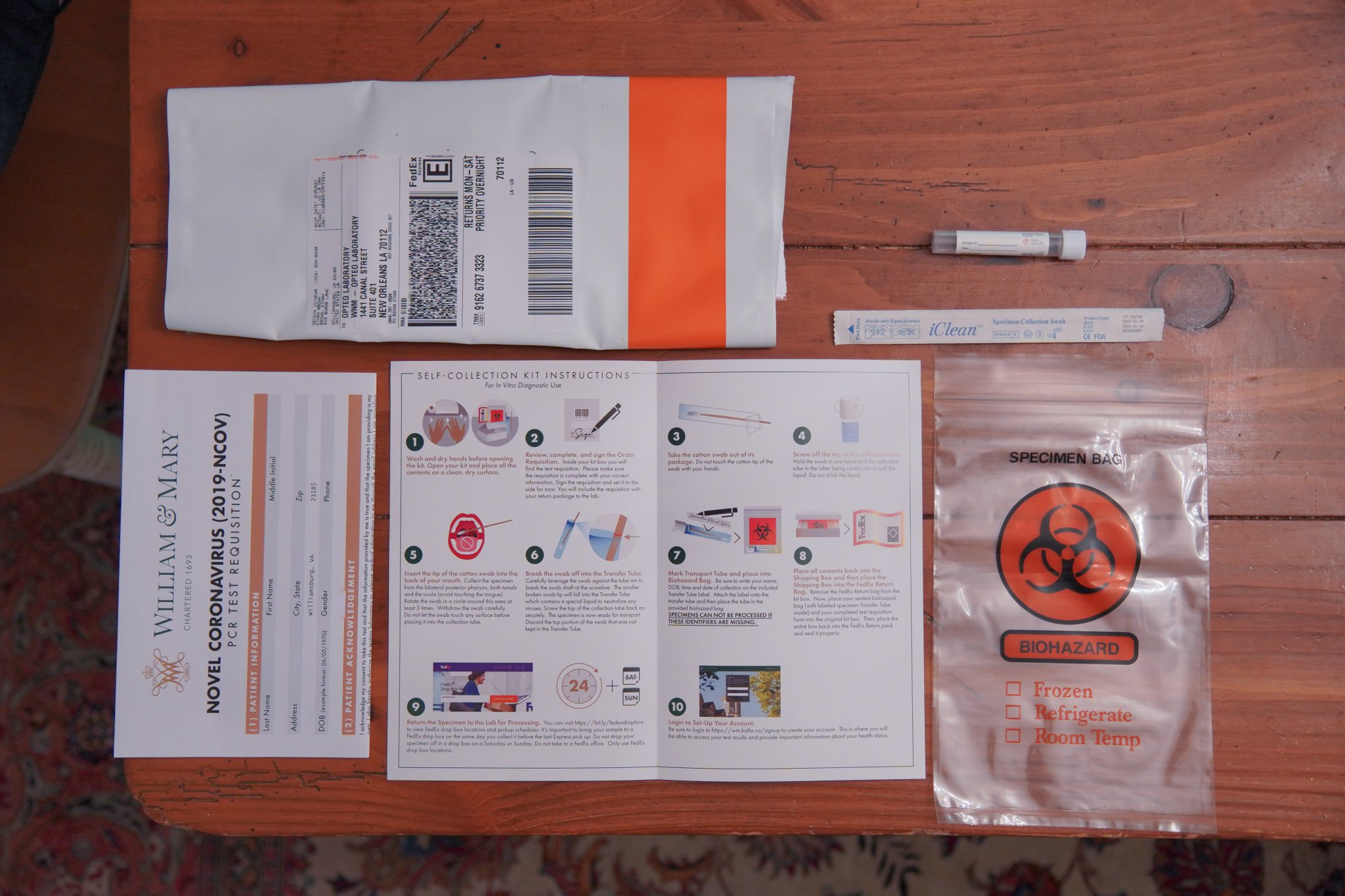In the image, on the left side, there is a piece of paper positioned sideways with bold black text reading "Novel Coronavirus 2019-nCoV". Above this text, "William and Mary" is written. Below this header, the paper has several rows of text alternating between white and gray backgrounds, though the text is too small to read clearly.

To the right of the paper, there is an open guide that lays out ten steps on what to do. These steps are labeled with white numbers inside black outlined circles. The guide spans across the page with steps 1 and 2 at the top left, steps 3 and 4 continuing across horizontally, and so forth.

Above the guide, there is a barcode typically used by FedEx or another mail system, along with tracking information and an address. Adjacent to this, on the right side, there is a swab and a small white piece of paper. Below these items, a clear plastic bag with a biohazard symbol is visible, suggesting that this is a COVID-19 test kit intended for self-testing and mailing back after sample collection.